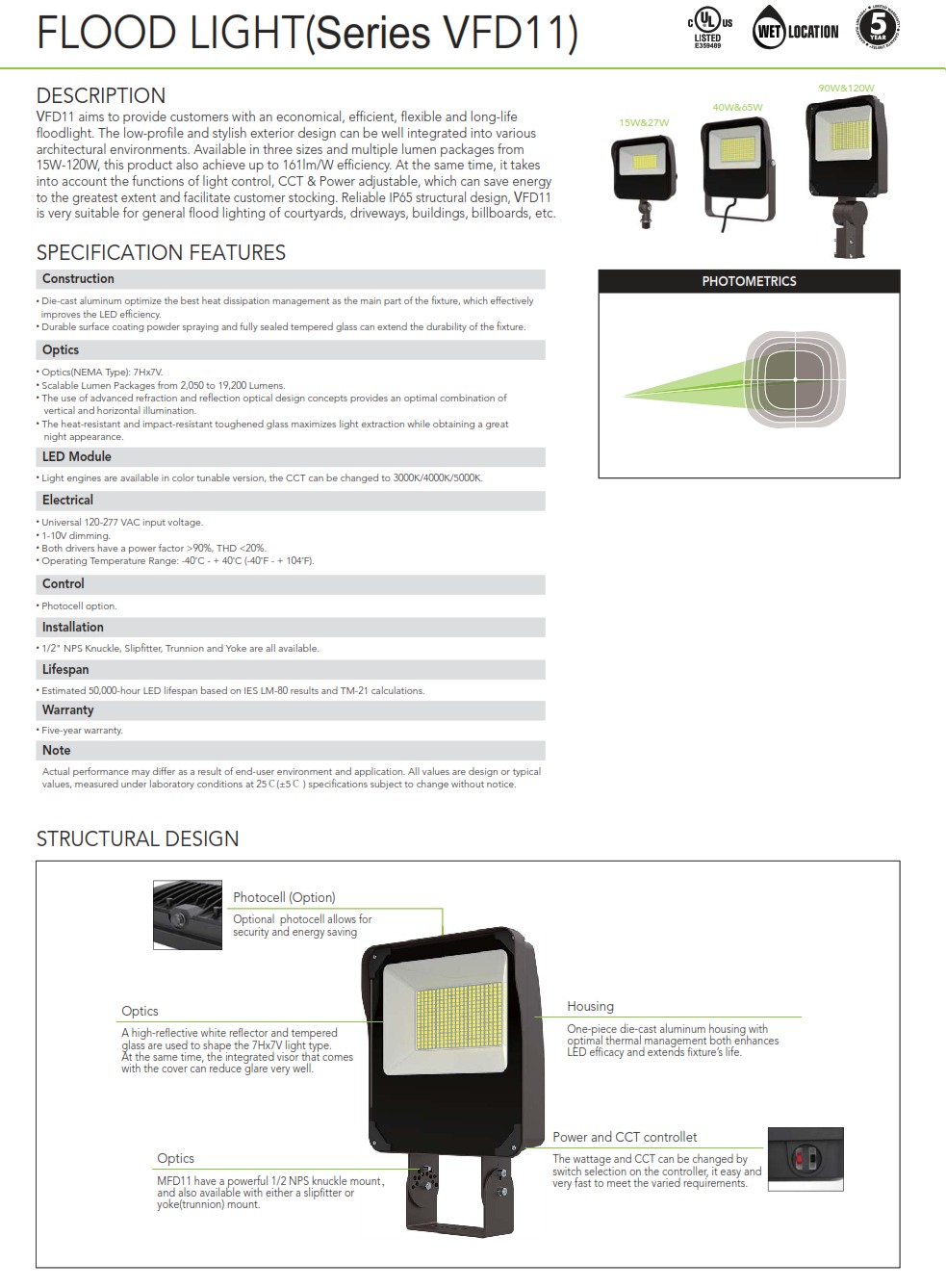This detailed product description page showcases the specifications and features of a floodlight. At the top of the page, the title "Floodlight" is prominently displayed, accompanied by the series number in parentheses to the right. Adjacent to the title are three distinctive logo icons. A green bar divides the header from the main body of the form.

Immediately below the green bar, the section titled "Description" provides a comprehensive paragraph detailing the floodlight. Following this, the "Specification Features" section is laid out with bullet points categorizing information under headings such as connection, LED module, electrical, control, lifespan, and warranty type.

On the top right, three product images and a detailed diagram offer visual references. The bottom of the page is dominated by a substantial section labeled "Structural Design." At the center of this section is a thumbnail of the product, with lines radiating out to descriptions of each specific feature, providing a clear and thorough understanding of the floodlight's structural components.